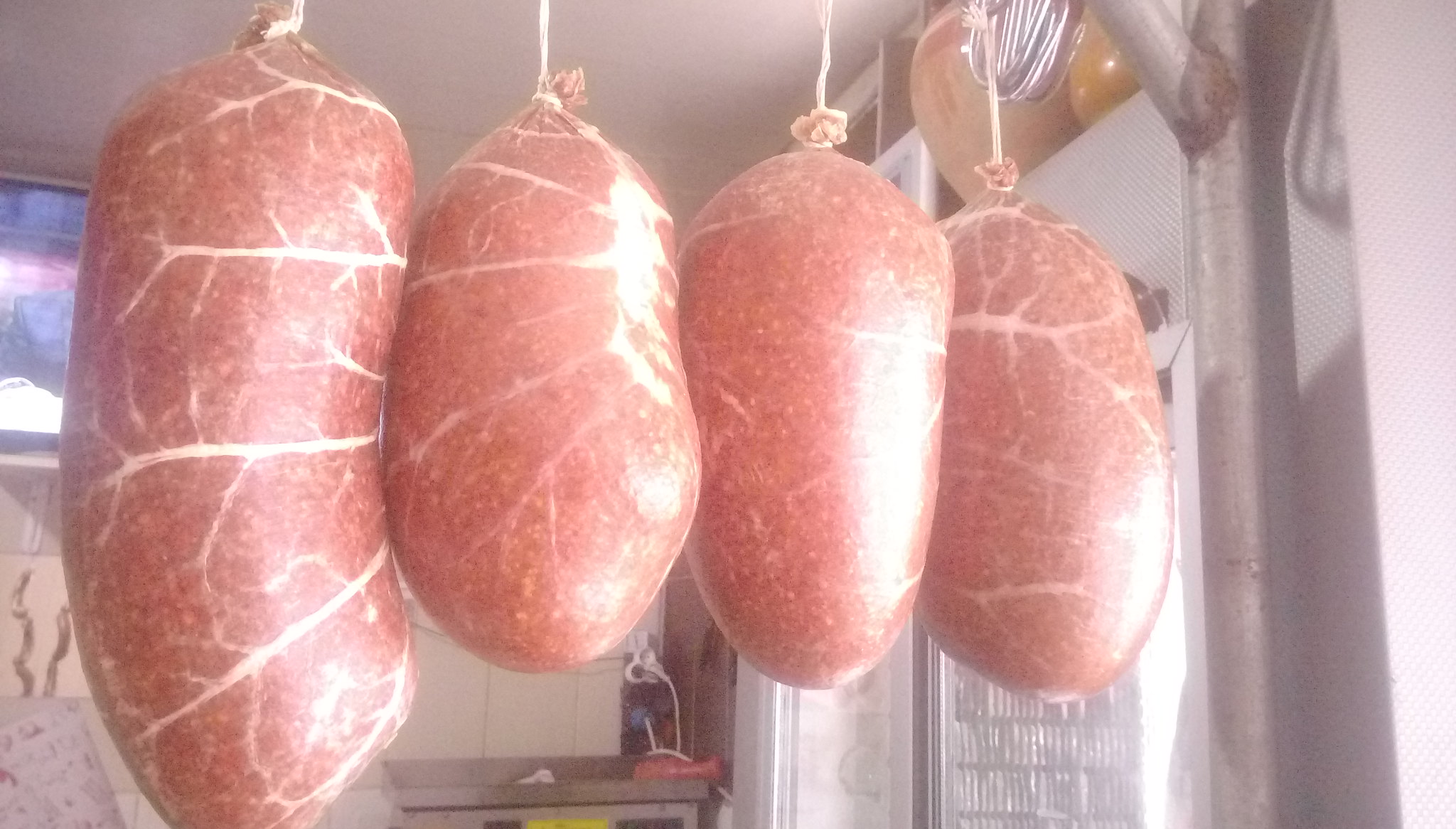The image depicts a somewhat unsettling scene inside what appears to be a butcher shop or kitchen, characterized by white tiled walls typical of such environments. The ceiling is also white, contributing to the stark atmosphere. On the right side of the image, there is a glass partition or window. In the background, a television screen glows, adding to the otherwise clinical setting. 

Central to the image are four large, somewhat indistinct blobs of meat hanging from a metal pole that cuts across the frame. This pole stretches from the right side, just above a visible metallic surface, and extends towards the left. The meats are encased in a casing resembling stretched intestines, with some pattern suggesting they might be tied with strings at the top to hold their shape. They're varying in size and shape—a large round one to the far left, followed by a smaller, jellybean-shaped one, and two more medium-sized pieces. The photo is slightly blurry and muted in color, perhaps due to a dirty lens, giving it an eerie, almost antiquated feel. The overall environment hints at a refrigerated or freezer area, emphasized by the bright lighting and somewhat cold atmosphere.